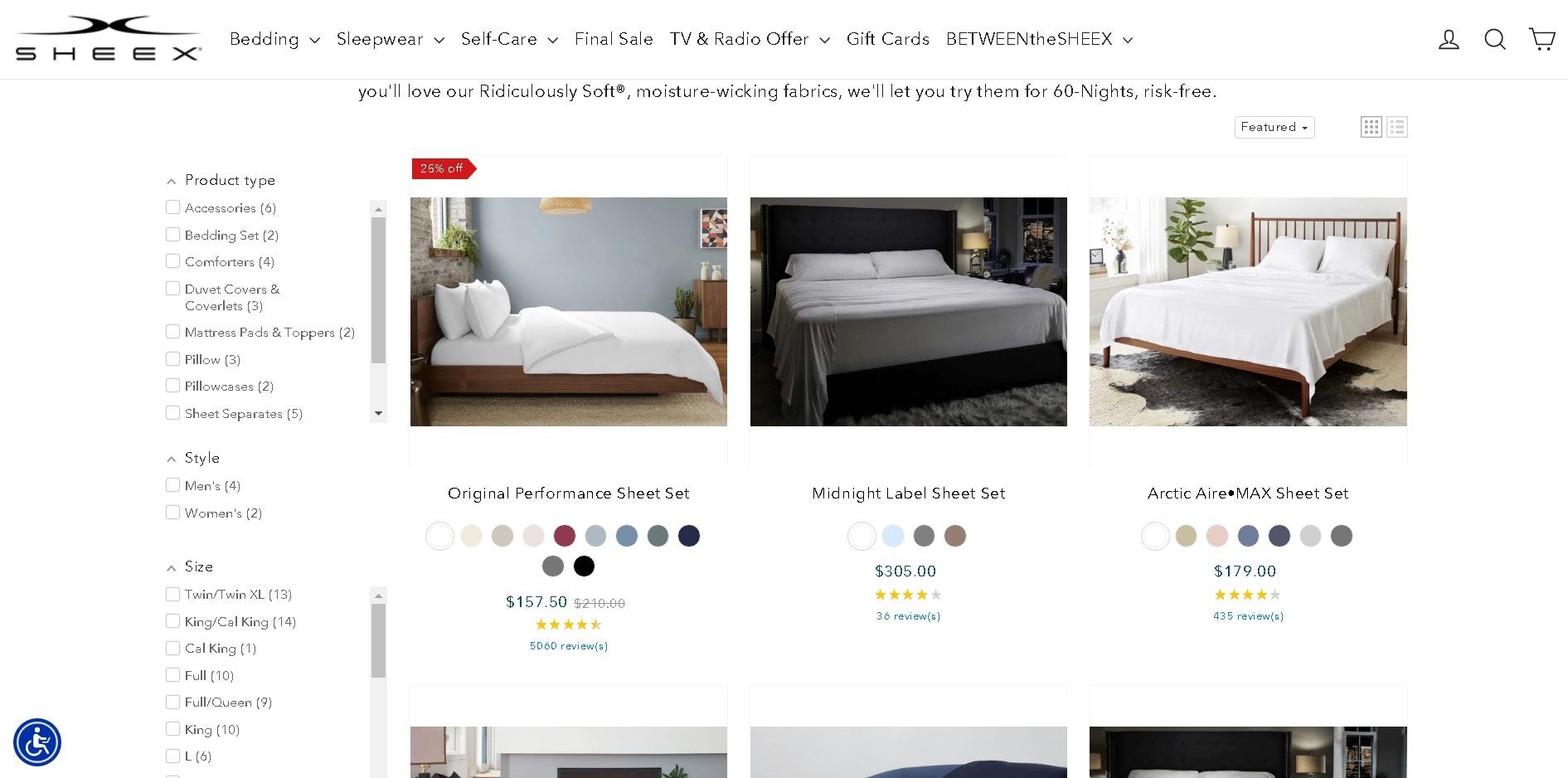Here's a cleaned-up and detailed caption for the image:

---
The image has a white background featuring various promotional elements for SHEEX bedding and sleepwear, emphasizing self-care and special sales. In the upper left corner, there is a text box highlighting the promotional offers: "Final Sale," "TV and Radio Offer," and "Gift Cards." Additionally, it mentions, "Between the Sheets," with a tagline: "You'll love our ridiculously soft, moisture-wicking fabrics. Try it for 60 nights risk-free."

Below this, three pictures of neatly made beds are placed side-by-side, showcasing different bedding sets. 

- The left image displays the "Original Performance Sheet Set," priced at $157.50.
- The center image features the "Midnight Label Sheet Set," priced at $305.00.
- The right image shows the "Arctic Air Max Sheet Set," priced at $179.00. 

On the left side of the image, there is a sidebar that lists various product types, including "Accessories," "Bedding Set," "Comforters," "Duvet Comforters," "Mattress Pad," "Toppers," "Pillows," "Pillowcases," "Men's," and "Women's."

The overall layout is clean, and the text effectively highlights the products and benefits of SHEEX bedding.
---

This caption provides a clear and comprehensive description of the image, capturing all essential details.